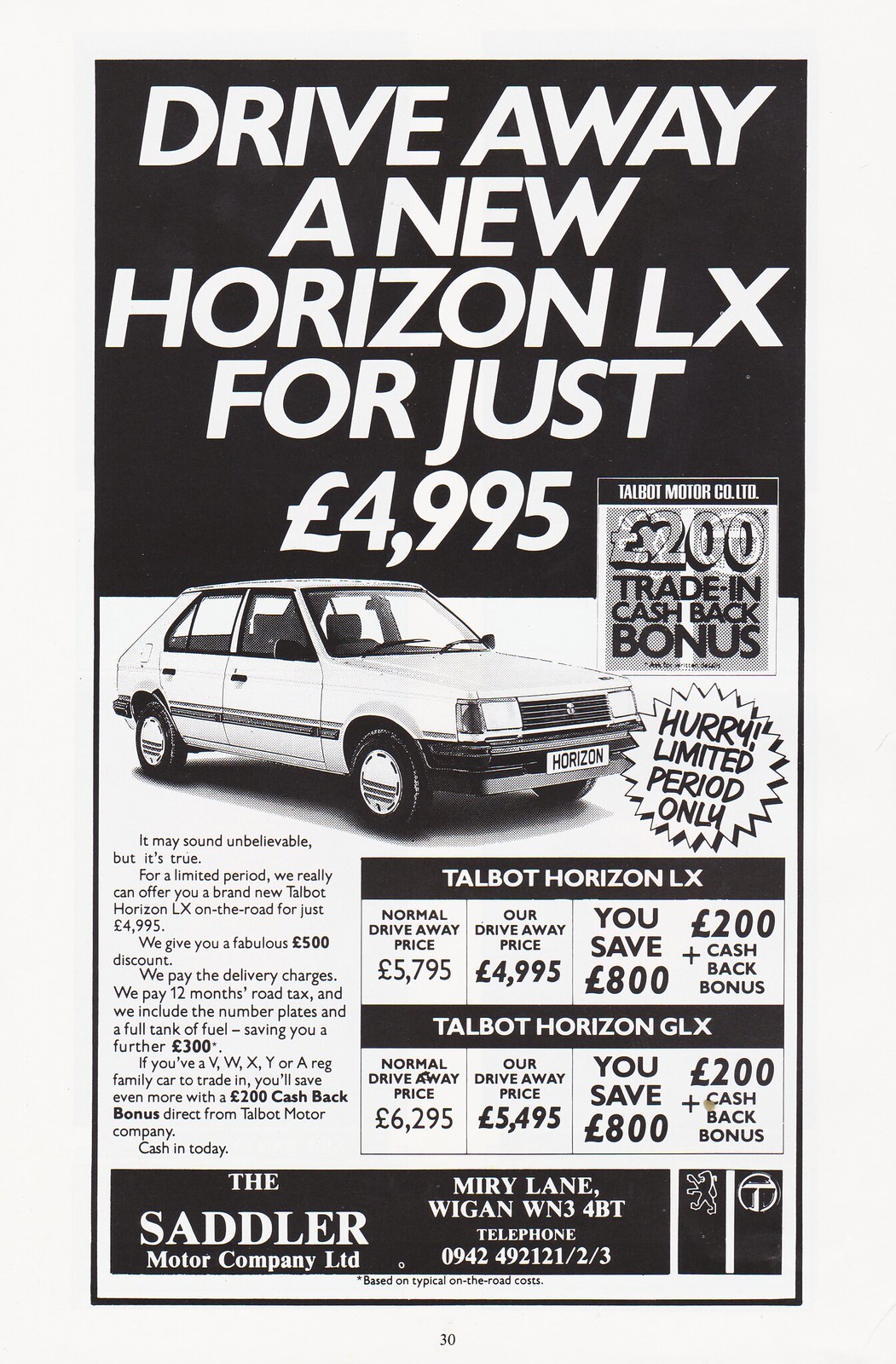This image is an advertisement for a car, featuring a retro black, white, and gray theme, reminiscent of the 1970s or 1980s. The ad is a tall rectangle with a white border. The top third has a black background with white italic text stating, "Drive away a new Horizon LX for just 4,995 euros." Beneath this, occupying the bottom third, is an image of a small white Talbot Horizon LX car set against a white background. To the left of the car are several paragraphs in black text detailing the offer: a limited-time deal providing a brand new Talbot Horizon LX for just 4,995 euros, inclusive of a 500 euro discount, delivery charges, 12 months road tax, number plates, and a full tank of fuel which collectively save 300 euros. An additional 200 euro trade-in cashback bonus is offered for VWXY or REG family car owners, making the total savings up to 800 euros. To the right of the car image, the ad presents pricing information for two Talbot models: the Horizon LX and GLX. The normal and discounted prices are shown, highlighting the 800 euro savings. At the very bottom of the ad, dealership information for The Sadler Motor Company Limited is provided, including contact details and a small number "30" that likely indicates a page number.